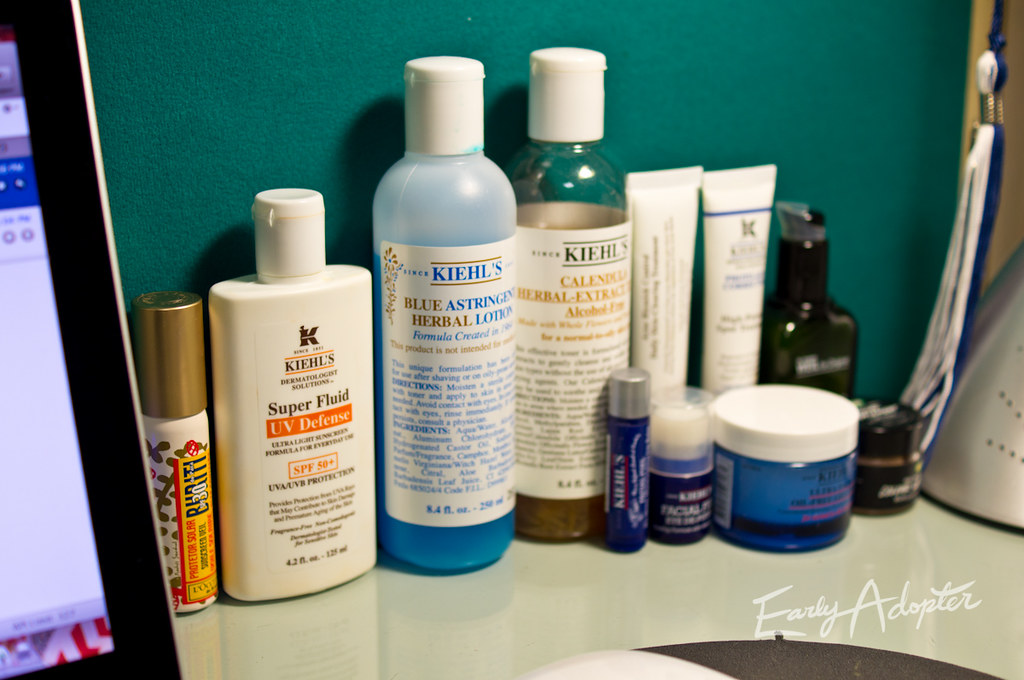The image depicts a well-organized bathroom countertop or possibly a workstation, laden with an array of skincare products. Prominently displayed in the bottom right corner is the phrase "Early Adopter," written in white text. On the left side of the image, a white tablet is visible, presumably next to a small white bottle with a gold cap, possibly containing balm. The countertop features various Kiehl's products, including a Superfluid UV Defense SPF 50+ sunblock and a blue astringent herbal lotion. 

Towards the back right, there are two white bottles standing beside each other, while in the bottom right corner, there are multiple blue bottles of different sizes, all with white caps. Additionally, the presence of black objects in the background and a monitor on the left side suggest that this could either be a bathroom or a professional workstation, such as a doctor's office. The word "Tacit" can be seen on the right side of the image, adding another layer of context to the setting filled with numerous lotions and skincare items.